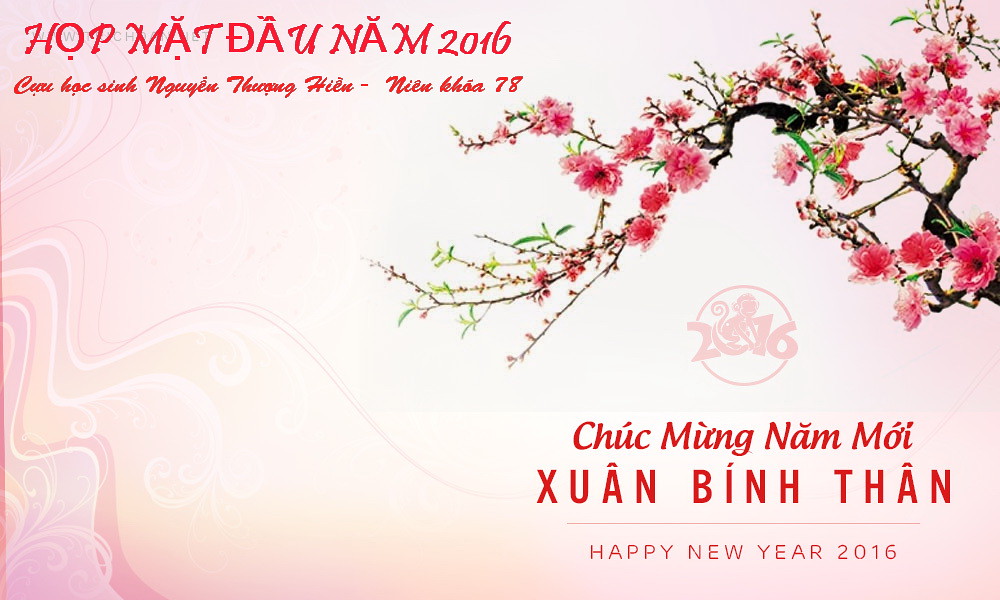The image is a digital graphic collage with a light pinkish-orange swirly background, featuring wavy lines intermingling in shades of light pink, beige, and white that run through the lower and upper left-hand corners. Dominating the upper right corner of the image is a narrow tree branch adorned with vibrant green leaves and delicate pink flowers. In the top region, red text reads "Hộp Mạt Đuôn Nam 2016," with additional details "Ninh Qua 78" beneath it. Below the blooming branch, there's a circle containing the number "2016" alongside the image of a monkey, symbolizing the Year of the Monkey. Further text below the circle says "Xu Cực Mưu Nam Mới Dương Bình Thành." A horizontal separator follows, with the greeting "Happy New Year 2016" completing the celebratory theme, indicating a New Year celebration graphic for the year 2016.